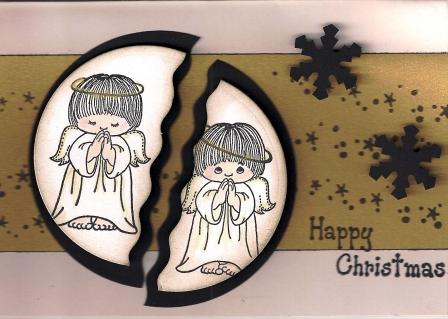In this digital image, set against a solid white background, a prominent gold stripe runs vertically through the center, adorned with black snowflakes of various sizes—two large ones on the right and smaller ones scattered around. In the bottom right corner, in a handwritten style, the words "Merry Christmas" appear in black. Central to the composition is an eye-catching illustration of a broken Oreo-like cookie. This cookie, split in half with a zigzag line, reveals two cartoonish, angelic boys within each half, each with big round heads, white robes, and gold halos. One angel has its eyes closed, while the other has its eyes open, both appearing to pray. The overall style of the image gives a handmade, homemade vibe, integrating white, tan, black, and off-green colors to create a festive, Christmas-themed visual.